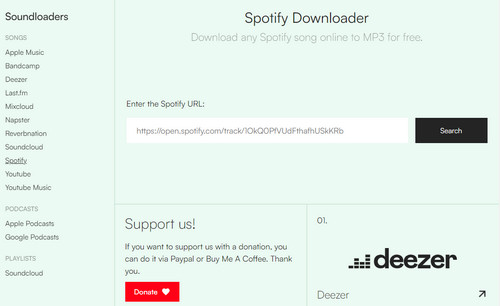The image is a screenshot of a downloader service interface titled "Soundloaders." At the top left corner, "Soundloaders" is prominently displayed. Directly below, a menu of various supported services is visible, including "Songs," "Apple Music," "Bandcamp," "Mixcloud," "Napster," "ReverbNation," "Soundcloud," "Spotify," "YouTube" (mistakenly read as U2), "YouTube Music," "Apple Podcasts," and "Google Podcasts." The central section of the screen showcases instructions, stating "Download a Spotify song" for free. Beneath this instruction, there is an input bar for inserting a URL, accompanied by a "Download" button. Additionally, there is a link for SSH access, likely for advanced settings or alternative download methods. At the bottom of the interface, there is a "Support Us" section with a link for donations, encouraging users to contribute financially to support the service.